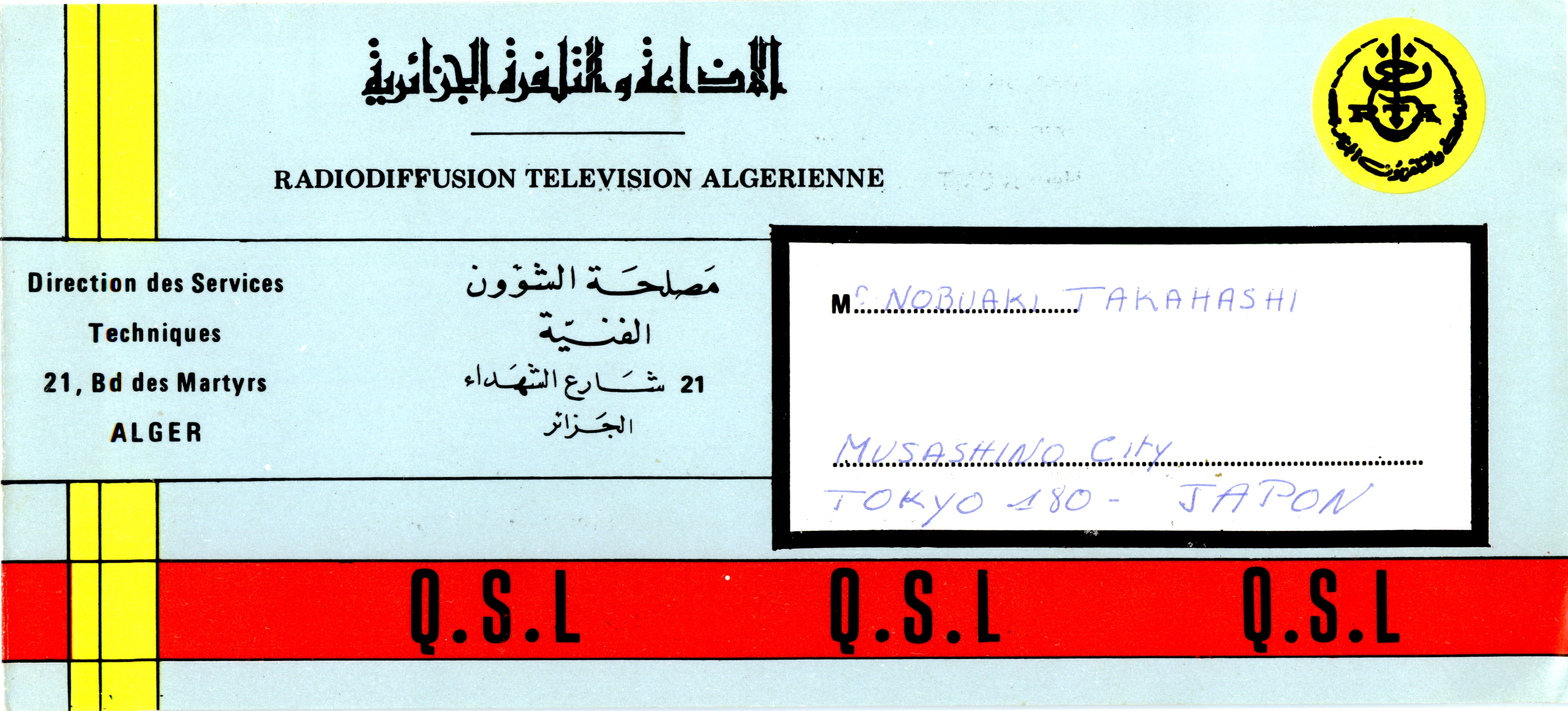This image is a dated QSL card from Radio Diffusion Television Algerian, likely used for official notifications in the radio and television industry in Algeria. The card is rectangular and light blue, featuring a vertical yellow stripe on the left side and a horizontal red stripe at the bottom, intersecting to form an overlap. At the top, Arabic script is present, alongside the words "Radio Diffusion Television Algerian." Below this, a blue bar reads "Direction Des Services Techniques, 21 BD Des Martyrs, Alger," with accompanying Arabic text. In a bordered white box, the letter "M" is printed, followed by a handwritten name in blue pen, "Nobuaki Takahashi." Beneath is a dotted line with the address "Musashino City, Tokyo, 80 Japon," indicating its recipient. A yellow seal is located in the top right corner, while the red stripe at the bottom bears the repeated abbreviation "QSL" in black, suggesting the card confirms the receipt of a radio signal.